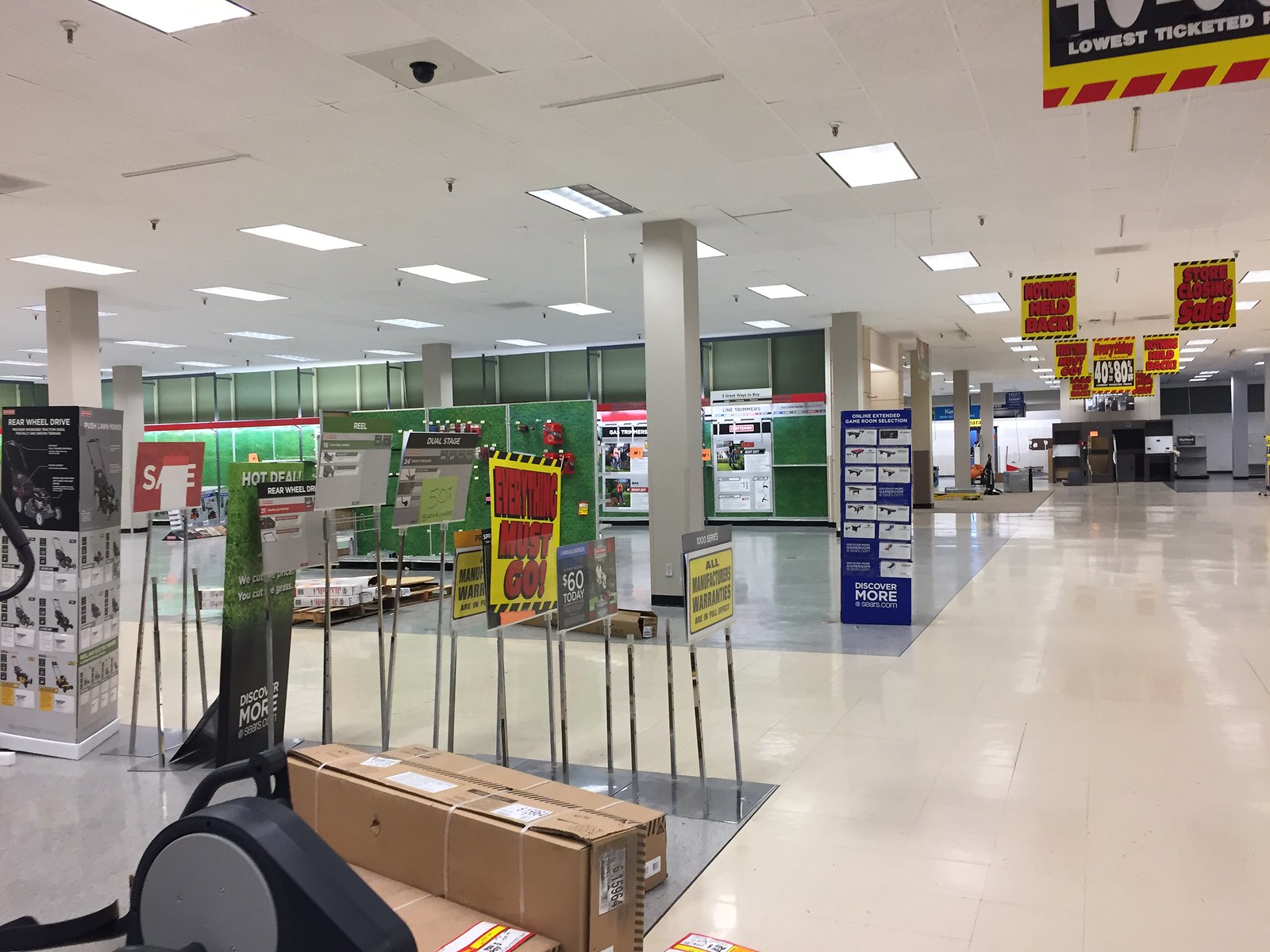This is a detailed photograph inside a large retail space, possibly a big box store, seemingly during a closeout sale as indicated by multiple "Everything Must Go" signs. The store, largely empty, features a classic white-tiled ceiling with rows of rectangular luminescent lights running diagonally from the left towards the far right, creating a diminishing perspective towards the back. Three prominent yellow banners with black trim and red lettering hang from the ceiling, reinforcing the sale message.

The floor is a combination of white and gray, segmented by square support beams scattered throughout the space. On the left-hand side, a row of green shelves holds various sale posters and advertisements, yet they appear almost entirely bare, suggesting a significant sell-out. In the background, likely near the far wall, a pile of boxes is stacked up but difficult to see clearly due to the distance.

In the lower portion of the image, particularly on the left side, several large, long rectangular brown cardboard boxes are visible, some secured with straps. Additionally, there's a black and gray machine that resembles part of an exercise bike, positioned near these boxes. The otherwise sparse scene is dotted with sale signage across the empty shelving and displays, reinforcing the store's ongoing clearance efforts.